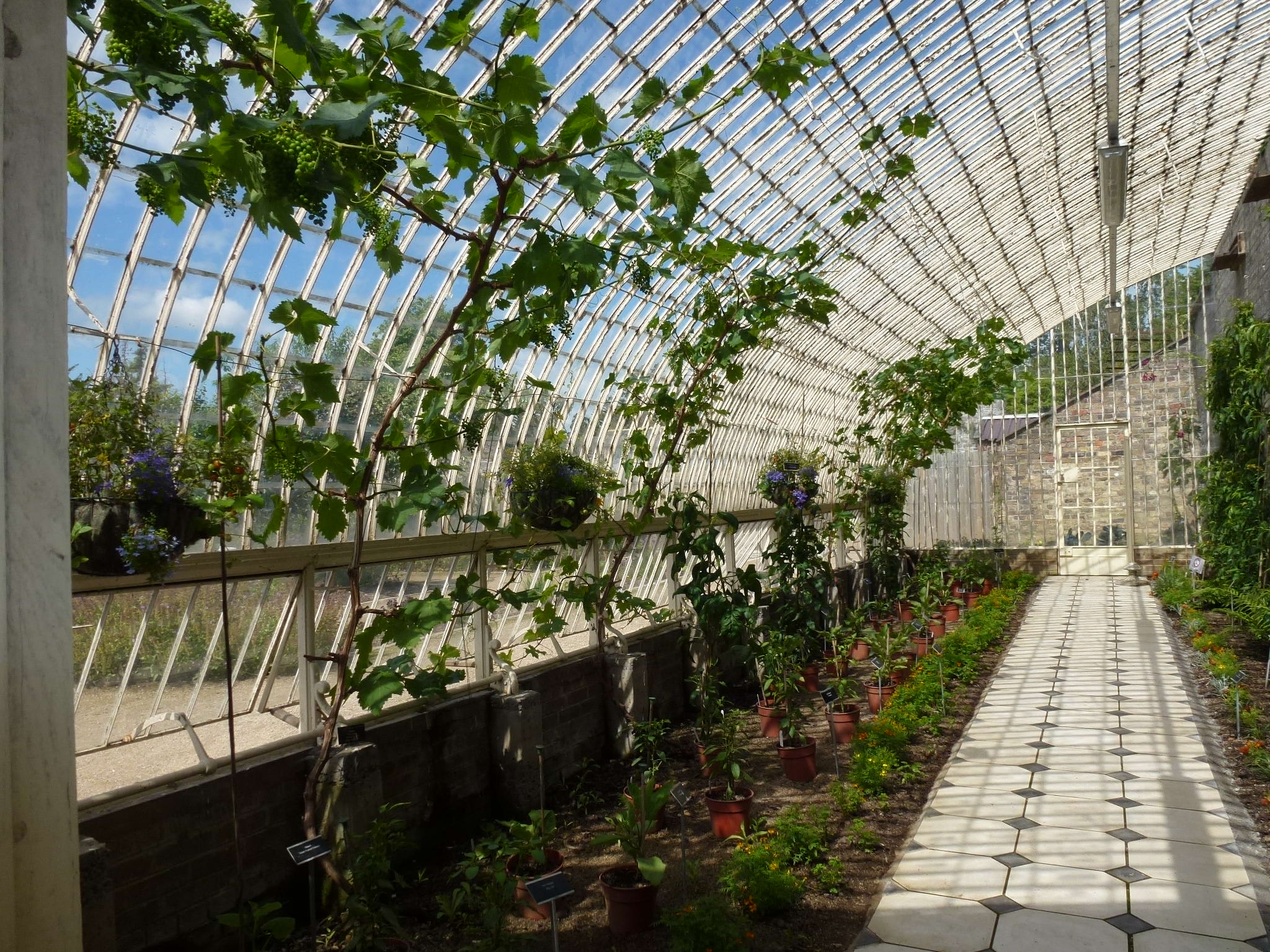This photo captures the interior of a conservatory greenhouse with an elegant, curved design. The greenhouse features arched glass windows that stretch from the ground up to the ceiling, allowing a clear view of the blue sky outside. A distinctive white and black diamond-patterned walkway runs from the bottom right through the center, leading to an exit door. The path is flanked by rows of lush green plants, some climbing high and others nestled in clay-colored pots, with a variety of small bushes planted directly into the brown soil. Sunlight streams through the glass, casting intricate shadows on the tiled walkway and soil below. In the backdrop of this verdant space, a brick building is visible, suggesting an adjoining natural area where additional plants or supplies may be stored. The entire scene is devoid of people, highlighting the serene, orderly beauty of the greenhouse.